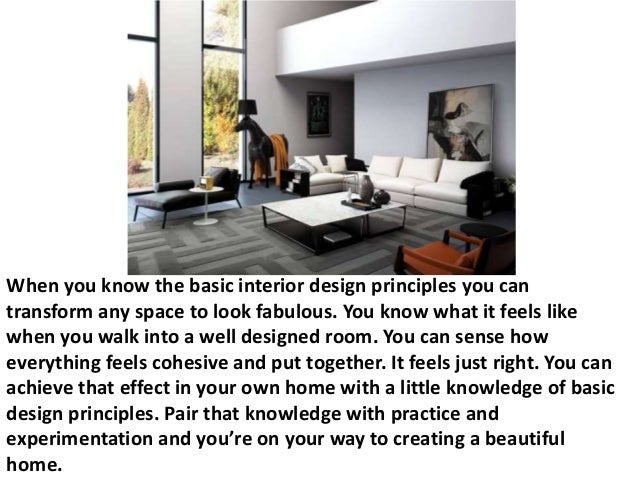This image depicts a modern, spacious living room with substantial natural light streaming through large, partially visible floor-to-ceiling windows. Dominating the space is a white sectional L-shaped couch with contrasting black arms and sides. The room is styled with sharp, clean lines and angular furnishings, including a sleek white coffee table and a small black lounger. A striking dark gray and light gray area rug adds texture to the otherwise smooth wooden floor. The walls are crisp white and adorned with a couple of paintings, adding subtle artistic touches to the room. Near the hallway stands a black horse sculpture, complemented by a brown chair and a lamp, which creates a stylish, cohesive vignette. Below the image is a black-font caption on a white background, emphasizing the transformation achievable through basic interior design principles, advocating for knowledge, practice, and experimentation to create a cohesive and fabulous home environment. This layout exudes a balanced, well-designed feel, akin to an advertisement for an interior design company.